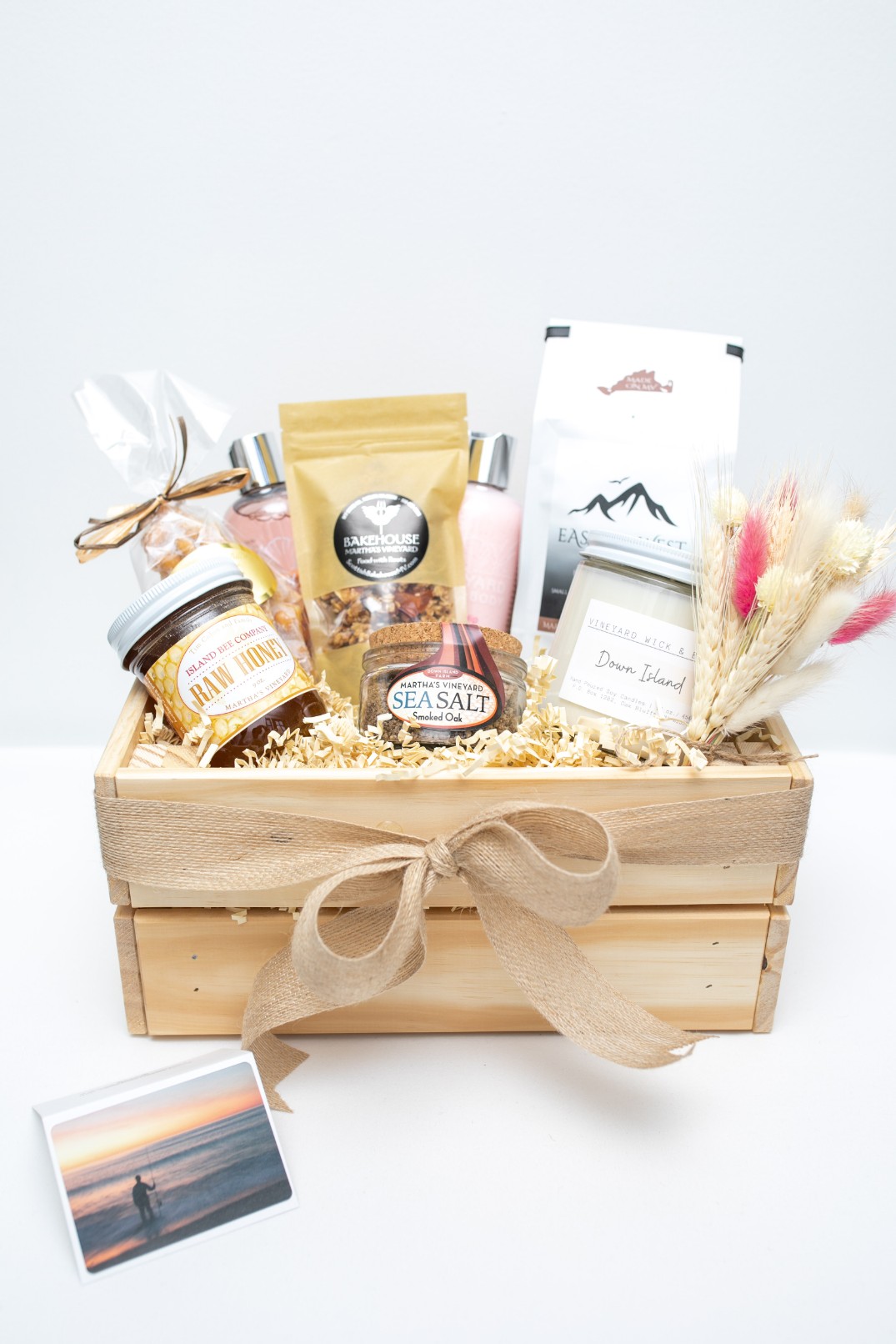The image is a professionally photographed, close-up shot of a mildly rustic yet elegant gift basket set against an all-white background. The gift basket, housed in a beige wooden crate, is adorned with a homespun burlap ribbon tied in a bow. The interior is filled with crinkled, tan-colored filler paper, adding a natural touch.

Prominently featured in the front of the basket is a card displaying a serene scene of a person with a fishing rod standing in the ocean at sunset. This gives the basket a leisurely, coastal theme.

Inside the basket, on the left, there's a jar of raw honey with a silver metal cap, and behind it, a bag tied with a gold ribbon. Adjacent is a clear glass bottle with a cork lid labeled "sea salt," specifically from Martha's Vineyard, indicating a smoked oak and down island variety. A pink bottle with a metallic lid containing a pink liquid, likely a body wash or lotion, sits behind this.

The center of the basket holds a package labeled as bakehouse snack mix, while to the right, a bundle of pale bone-colored thistle flowers and pink ones adds a decorative, organic element. Near this, there's a white jar possibly containing a candle, resembling a Yankee Candle. There's also a white package that might be coffee or similar, accompanied by another pink bottle of translucent liquid with a silver cap.

The assortment of items in the gift basket — including a candle, body wash, raw honey, sea salt, and snacks — alongside the sea-themed card, collectively convey a thoughtful, beach-inspired gift perfect for a variety of occasions.